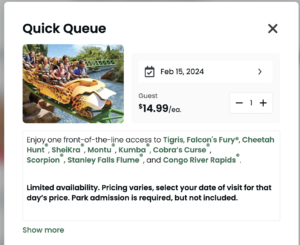The image is a screenshot from a website. The page has a thin border on the left, top, and right sides, with the top and right borders being particularly narrow. The webpage features a white background. 

At the top, prominent text reads "QuickQueue," with "QUICK" and "QUEUE" both in uppercase letters, and a large "X" symbol is positioned to the right. 

Beneath the title, there is an outdoor image that appears to depict a theme park scene with a roller coaster. The roller coaster is carrying several people, and below it, there is water, some trees, an island on the right side, and rocks on the left.

Following the image is a calendar icon with a checkmark, indicating the date "Feb 15, 2024," accompanied by a right-facing arrow. The text beside it reads "Guest $14.99/EA." Below this, there is a white square containing a minus sign, the number "1," and a plus sign, presumably for adjusting the quantity.

Further down, there is a description section with a "Show More" option highlighted in green text.